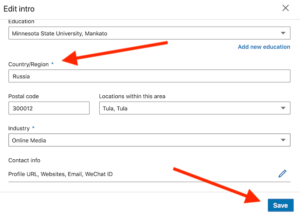This image is a screenshot of an editable form section. The background is white and it lacks any border. In the upper left-hand corner, the text "Edit Intro" is displayed, accompanied by a blue pen icon situated just above a blue "Save" button in the bottom right-hand corner. A red arrow points from the center of the form to the "Save" button.

In the top portion of the form, a dropdown menu is labeled "Education," with the current selection being "Minnesota State University." Below this, a new section reads "Country/Region," with "Russia" entered in the box. An adjacent red arrow draws attention to this field from the top scroll bar box.

Further down, additional boxes gather information such as postal code and specific locations within the selected region, which is specified as "Tula, Tula." Following this section, another scroll bar is labeled "Industry," containing the text "Online Media."

At the very bottom, contact information fields are provided, including options for Profile URL, Websites, Email, and WeChat ID. Another red arrow points from the form's center towards the "Save" button. The overall layout is designed for input and updating of personal and professional details in a structured manner.